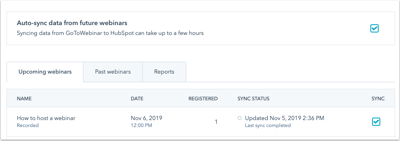This image showcases a settings page from an application or website, presented in a landscape orientation. The page is framed by a dark black border on the left and bottom, with a lighter gray border on the top and a slightly darker gray border on the right. The primary background is white, and the page's width is approximately double its height.

At the top of the page, a thin gray box spans horizontally, containing black text that reads, "Auto-sync data from future webinars." Below this, in gray font, there's a note stating, "Syncing data from GoToWebsite to HubSpot can take up to a few hours." To the right of this message is a small blue box with a white background, featuring a blue checkmark inside it.

Beneath this section, there are three tabs aligned horizontally across the screen: "Upcoming Webinars," highlighted in white; "Past Webinars," housed in a gray box; and "Reports," also in gray. Below these tabs, a header row lists column titles: "Name," "Date," "Registered," "Sync Status," and "Sync." The section below the header has a white background with smaller text. Under the "Sync" column, there is another blue box with a blue checkmark within it.

This detailed layout provides a comprehensive view of the sync settings and webinar management features within the application or website.